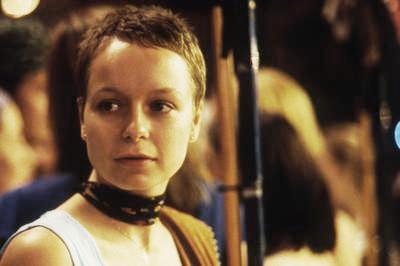The image captures a scene likely from a movie, depicting a young woman with a very short, pixie-cut hairstyle, somewhere between dirty blonde and brown. She is wearing a white tank top and a black choker or small scarf around her neck. Draped over her left shoulder is a brown garment, possibly a shirt. The background is blurred and features indistinct heads of people with varying hair colors—brown, blonde, and curly black—and what appear to be vertical poles or writing utensils. The overall lighting casts a light yellow glow, adding to the muted and slightly low-quality appearance of the photograph. The woman is looking slightly to the side, not directly at the camera.